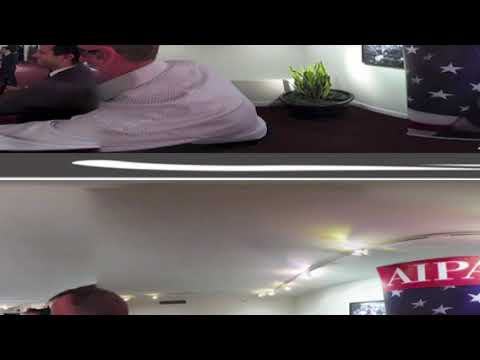The image depicts a somewhat distorted scene, seemingly split and inverted horizontally, where the top part appears at the bottom and vice versa. Dominating the image is a man with a red-tinted, demonic face wearing a white collar shirt, whose head is bizarrely displaced across the two halves of the picture. To his left, there is also a man dressed in a gray suit with short black hair, positioned against a backdrop that includes a poster with an American flag. Surrounding these figures is a room with white walls adorned with fluorescent lights and spotlights lining the ceiling edges. A green potted plant in a black pot is visible towards the top center of the image. A notice featuring "AIPA" printed in white against a red background along with a blue rectangle embellished with white stars is also discernible. The floor is brown, contrasting with the predominantly white interior. There is an additional black and white portrait on the wall, adding to the room's decor.